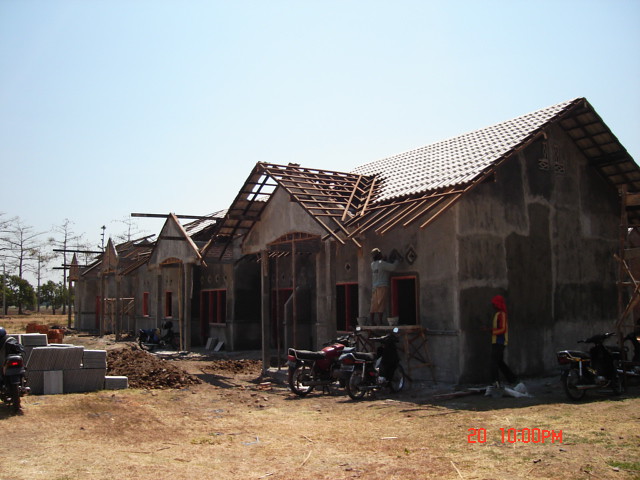This image captures a house under construction, set against a backdrop of a clear, bright blue sky devoid of clouds. In the distant background, there are two types of trees: some tall and leafless, and others shorter and green. The majority of the foreground consists of a dirt field. Dominating the scene is the half-finished house with its gray, unpainted exterior walls constructed from blocks. Unfinished brown wooden pieces are visible, forming part of the roof awning. 

Towards the right side of the building, a man wearing a light blue shirt and khaki pants stands on a raised platform, engaged in construction work. Near him is another individual, identifiable by a red hat and a striped jacket, walking towards the structure. Scattered in front of the house are four motorcycles: one in the upper left-hand corner visible side-on, two positioned centrally, and one on the far right. There's a construction material pile, possibly gray in color, located near the back of the motorcycle on the far left. The upper third of the photo is predominantly composed of the sky, with a timestamp reading "2010 PM" visible on the image.